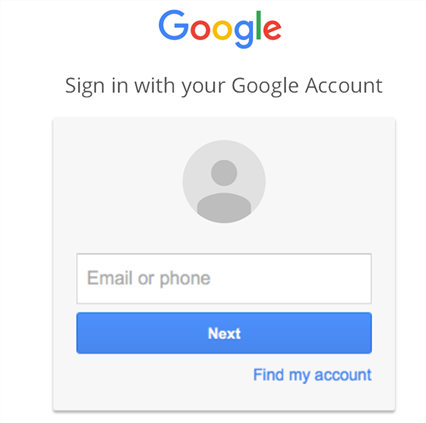The screenshot appears to be of a Google sign-in page, fitting within the dimensions of a large cell phone screen. At the top center, the Google logo is prominently displayed, featuring the signature colors of blue, red, yellow, green, and red. Beneath the logo, the prompt "Sign in with your Google account" is clearly visible.

In the middle section of the page, there is a placeholder profile icon—a generic silhouette consisting of a circle to represent the head and a partial oval below to represent the torso—set against a lilac-gray background commonly seen on devices. Directly underneath this icon, there is a white input bar labeled "Email or phone," inviting users to enter their credentials.

Further down, a prominent blue button labeled "Next" is positioned for user interaction. In the lower right quadrant, slightly above the blue bar's bottom edge, the text "Find my account" is displayed in blue, occupying an estimated two-thirds of the space horizontally.